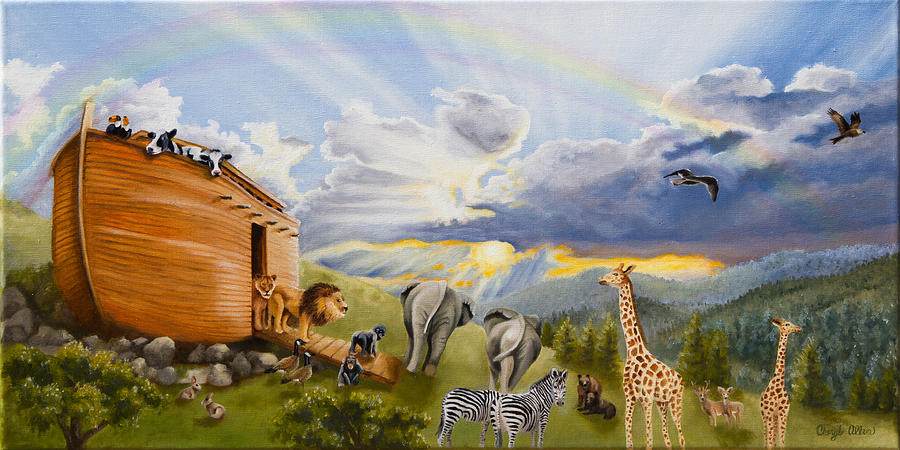This vibrant full-color painting, horizontally rectangular with no border, vividly depicts the scene of Noah's Ark post-flood. Dominating the center left is the Ark, its ramp door open, suggesting the animals are beginning to explore their new surroundings. The Ark is topped with a few toucans and cows peering over the edge. A pair of lions is prominently making their way down the ramp, while monkeys gather at its base. On the lush grass, a diverse array of animals, including ducks, bunnies, elephants, zebras, giraffes, deer, and bears, are scattered or wandering about. 

The sky is rich with clouds, and a faint rainbow stretches across, hinting at the subsiding storm. Behind the clouds, the sun casts a yellowish hue, illuminating the scene with a warm glow. Birds can be seen flying off towards the right. The landscape is verdant and thriving, adorned with green grass, trees, and distant mountains, enhancing the feeling of renewal and beginning. The lower right corner of the painting features a slightly blurry signature, attributed to the artist. The overall atmosphere of the image is bright and serene, capturing a moment of tranquility and hope after the catastrophic flood.